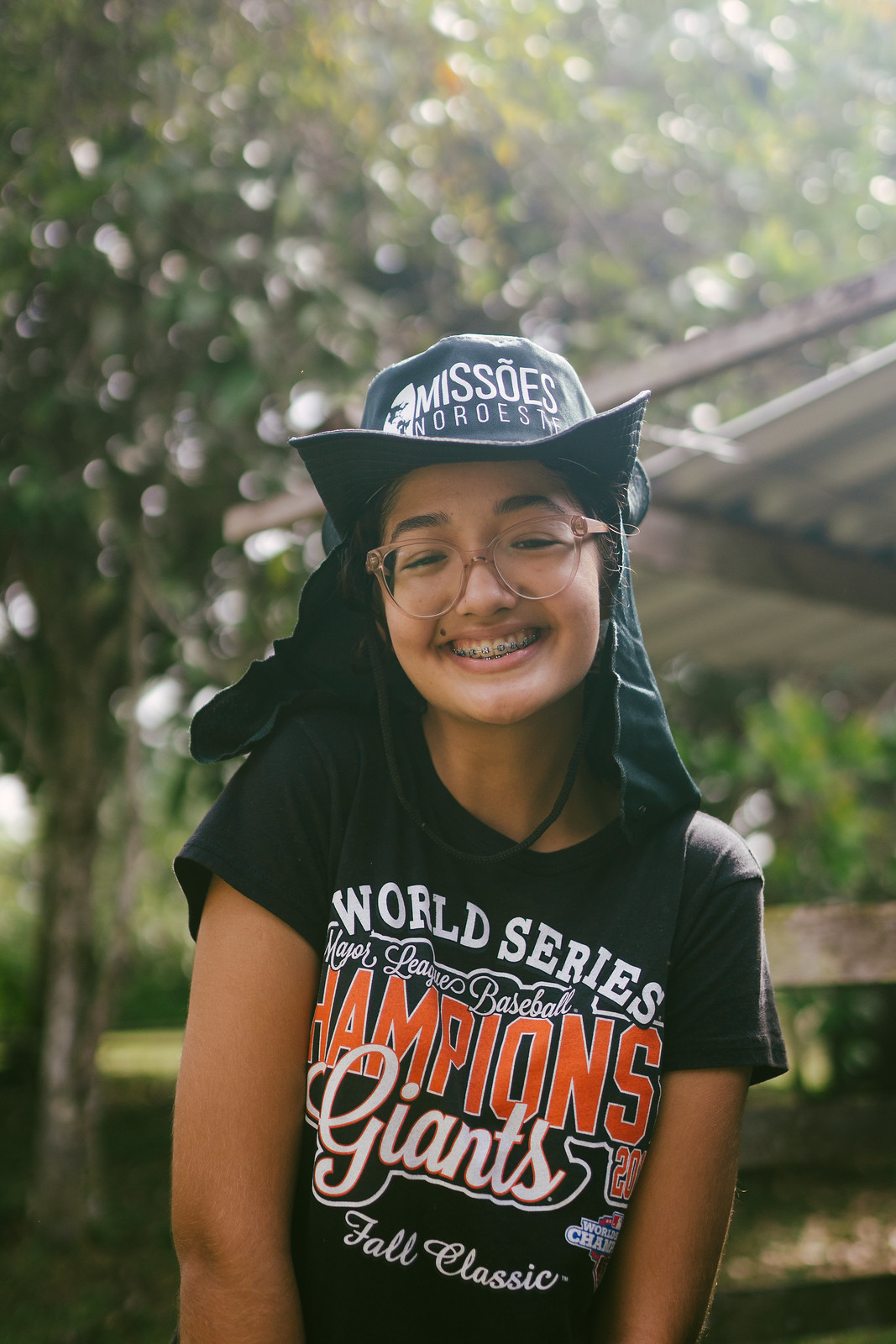The image captures an outdoor scene during the daytime, featuring a smiling girl with tanned skin who has blue braces. She wears large glasses and a navy blue hat styled like a parka or rain hat, with a string hanging around her neck. The hat has white lettering that reads "Missos" and "N-O-R-O-E-S," accompanied by a white logo. She is dressed in a black t-shirt that has several inscriptions: in white letters, it says "World Series," followed by "Major League Baseball" and "Champions" in bold orange letters with a white border. Below that, "Giants" and "Fall Classic" are also printed in white. The background shows a blurred view of greenery with several trees and a grass field, along with a wooden shelter or garage structure visible to the right.